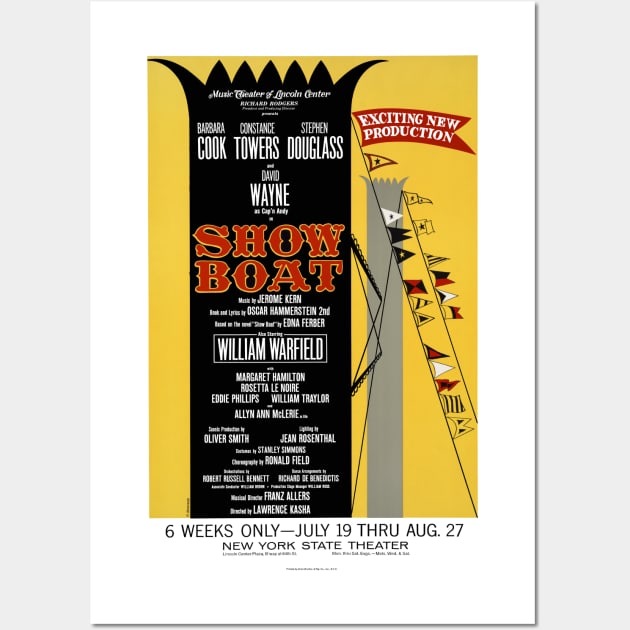This vibrant promotional poster for the event "Show Boat" is designed with a prominent yellow background. At the very top, a black, crown-like vertical strip features in bold white font, "Music Theater, Lincoln Center". Below it, the names Barbara Cook, Constance Towers, Stephen Douglas, and David Wayne as Captain Andy are also listed in white. The centerpiece of the poster is the event name "Show Boat", displayed prominently in bold red letters outlined in yellow.

Further down, additional details are provided in white text: "Music by Jerome Kern, Lyrics by Oscar Hammerstein II, based on the novel Showboat by Edna Ferber." The cast also includes William Warfield and Margaret Hamilton, along with Rosetta Lenoire, Eddie Phillips, William Traylor, and Aileen Ann McClure. Additional credits for sound production, lighting, and other roles are noted, but the text size decreases, making them harder to read. These names include Oliver Smith, Gene Ruhenthal, Stanley Simmons, Ronald Field, Robert Russell Bennett, Richard Debenix, Franz Ehlers, and Lawrence Kasha.

On the right side of the poster, a diagonal red pennant banner with white text proclaims "Exciting New Production". Attached to the banner pole are a series of multicolored maritime flags arranged in a line, adding a festive touch. Below the main yellow section, the poster announces in black text, "Six Weeks Only, July 19th through August 27th, New York State Theater." The overall design resembles a towering ship mast with flags, giving it a nautical theme that resonates with the title "Show Boat".